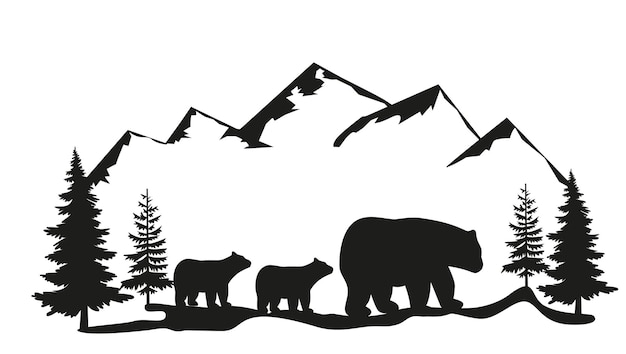The illustration is a detailed black and white pen and ink artwork depicting a serene woodland scene. At the top, five jagged mountain peaks are highlighted with precise black shadowing on their left sides. In the foreground, a thick, bold black line marks the ground. On the left lower corner stands a large pine tree silhouette casting a shadow to the right, accompanied by a smaller, less mature pine tree. Centered in the image are three bears: a larger adult bear leading the way with two smaller cubs trailing behind, all walking from left to right. Flanking the bears to the right are another set of pine trees, one small and one larger, completing the symmetrical composition of nature's tranquility.